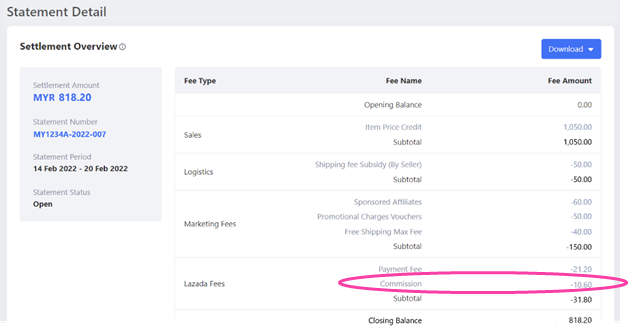The image features a document with a gray border. In the top left corner, the text "Statement Detail" is displayed. Adjacent to it, black text reads "Settlement," while a blue rectangle nearby says "Download." Immediately below, the document states the settlement amount as "MYR 18.20" and provides the statement number "MY1234A-2022-007." The statement period is listed as "14 February 2022 - 20 February 2022," and the statement status is "Open."

Continuing down, a table-like section provides detailed financial information. It includes columns labeled "Fee Type," "Fee Name," "Fee Amount," "Opening Balance," "Sale," "Item," "Price Credit," and other relevant headings. The opening balance is indicated as "0.00," followed by itemized entries such as:

- **Fee Amount**: MYR 1050  
  - **Fee Name**: Shipping Fee Subsidized by Seller  
  - **Subtotal**: MYR -50  
- **Sponsored Affiliates**: MYR -60  
- **Promotion Charges (Vouchers)**: MYR -50  
- **Free Shipping**: MYR -40  
  - **Subtotal**: MYR -150  

Additional charges are listed:
- **Payment Fee**: MYR -21.20  
- **Commission**: MYR -10.60  

A reddish-purple circle highlights a subtotal of MYR -31.80, and the closing balance is MYR 818.20. The background of the document is white, featuring various lines and columns to organize the financial details.